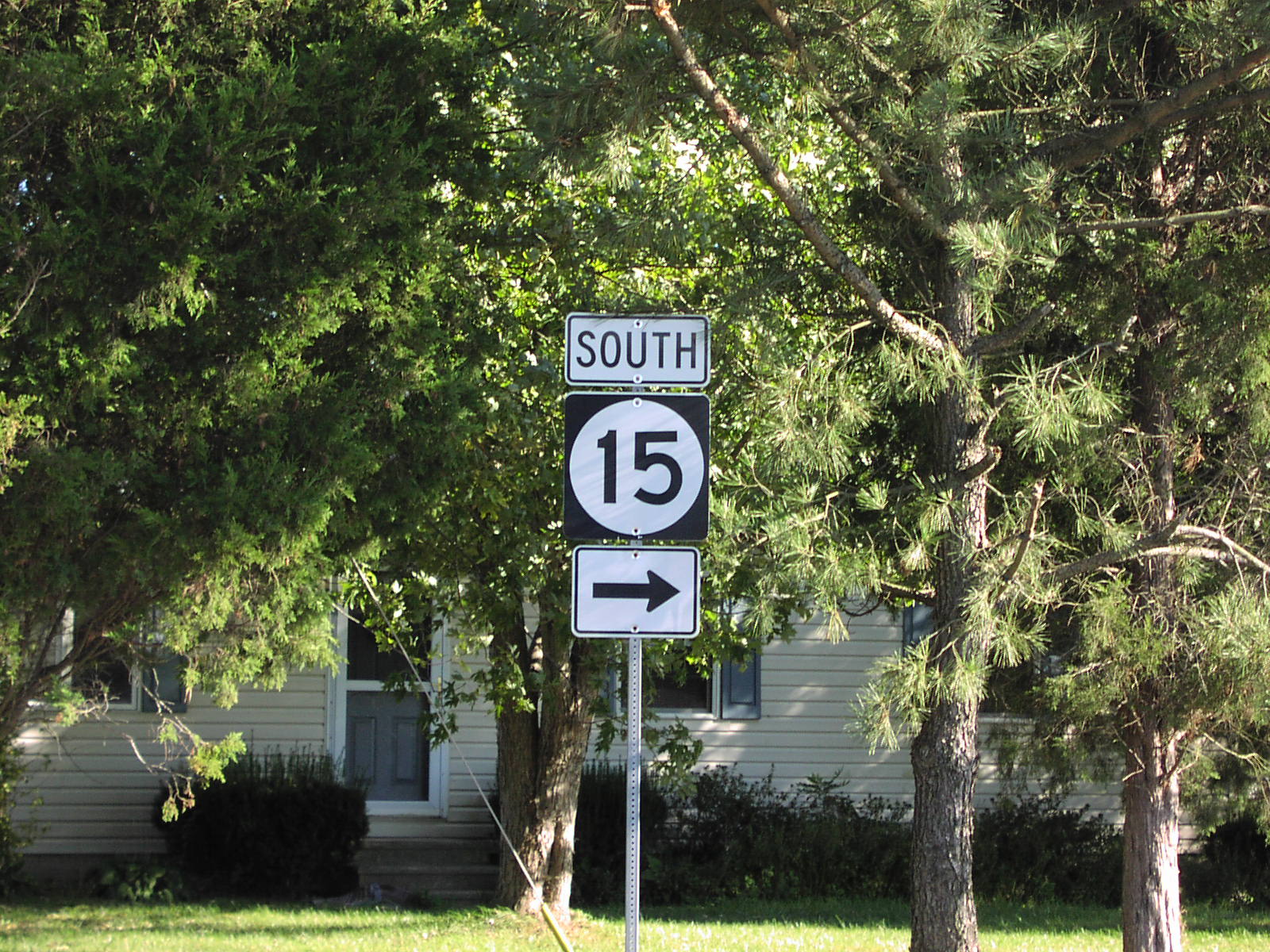On a bright and sunny day, an outdoor scene captures a picturesque house partially shaded by abundant greenery. The house features beige siding with greenish shutters adorning the windows, adding a charming touch. Multiple trees, including a couple of tall pines and an oak, stand prominently in the front yard, providing ample shade. The well-manicured lawn is neatly cut and partially shaded by the trees. Three steps lead up to the entrance of the house, which is bordered by well-maintained shrubberies. A street sign positioned at the front of the house reads "South 15" with an arrow pointing to the right, the number enclosed in a white circle with black lettering.